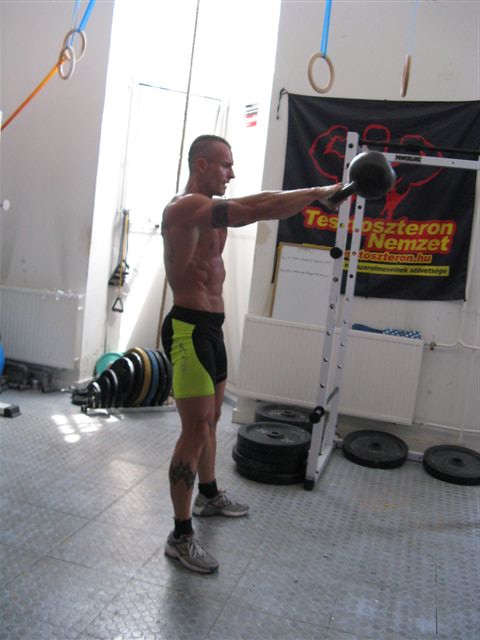The photograph captures a shirtless, well-toned man with a muscular build and a buzzcut, performing a kettlebell exercise in a modest gym setting, likely a personal gym due to its utilitarian appearance. He stands on a floor made of old metal panels or gray sectioned tiles, balancing with his legs slightly spread apart. He lifts a kettlebell in front of him, arms outstretched. The man's attire includes short black socks and neon green and black shorts that extend to his thighs, revealing his strong legs and tattoos on his arm and leg. 

In the background, the gym's details emerge: metal weight plates and barbells stacked and lined up near the walls, accompanied by various hanging equipment, such as blue bands connecting to rings and an orange rope. A black banner on the wall carries the word "testosterone" among other smaller, unreadable text. The gym space is partly illuminated by light from what could be a window. Additionally, a white weight lifting bench is visible behind the man, complementing the utilitarian ambience of this workout area.